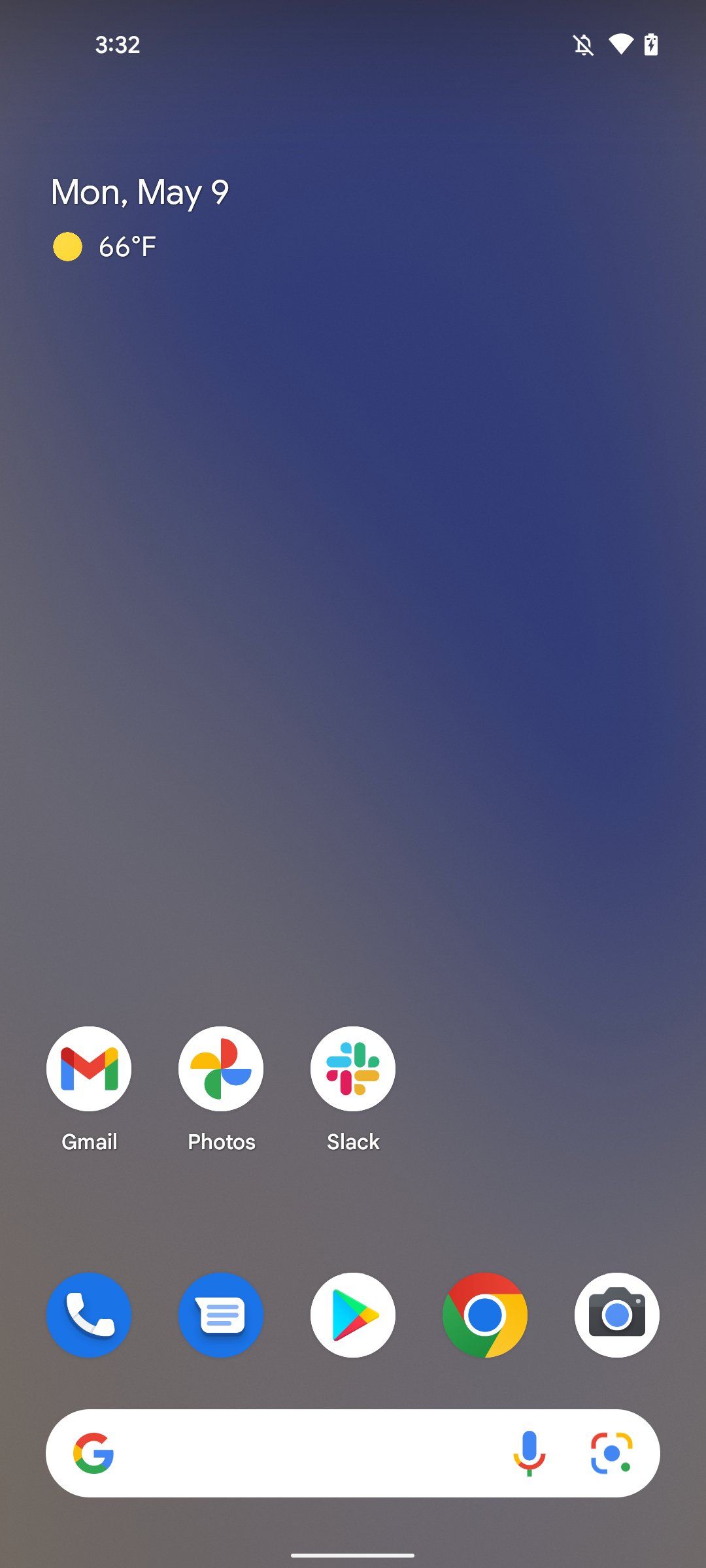A detailed image caption for the described scenario:

The image depicts the home screen of a smartphone, likely turned on and currently displaying various details. The background appears dimly lit, enhancing the visibility of the on-screen elements. At the very top, the date and time are displayed: "Monday, May 9th," alongside the current temperature, "66 degrees Fahrenheit," with a yellow sun icon indicating sunny weather. On the top left of the screen, the time "3:32" is clearly visible. Adjacent to this, on the top right, there are multiple status icons, including an indication that the volume is off and other icons suggesting power and connectivity status.

Dominating the bottom portion of the screen is a prominent white search bar with a colorful "G" representing Google on its left side, a microphone icon to its right, and a camera icon adjacent to that. Just above this search bar, there are five circular app icons in a horizontal row. From left to right, these icons represent a Phone app (blue icon), a Messaging app, a word processing app, Google Chrome, and a Camera app. Further upward, but still in the lower portion of the screen, there are three additional app icons for Gmail, Photos, and Slack, suggesting easy access to these applications.

A thin white line runs horizontally along the bottom edge of the screen, situated just below the Google search bar, adding a clear delineation to the layout.